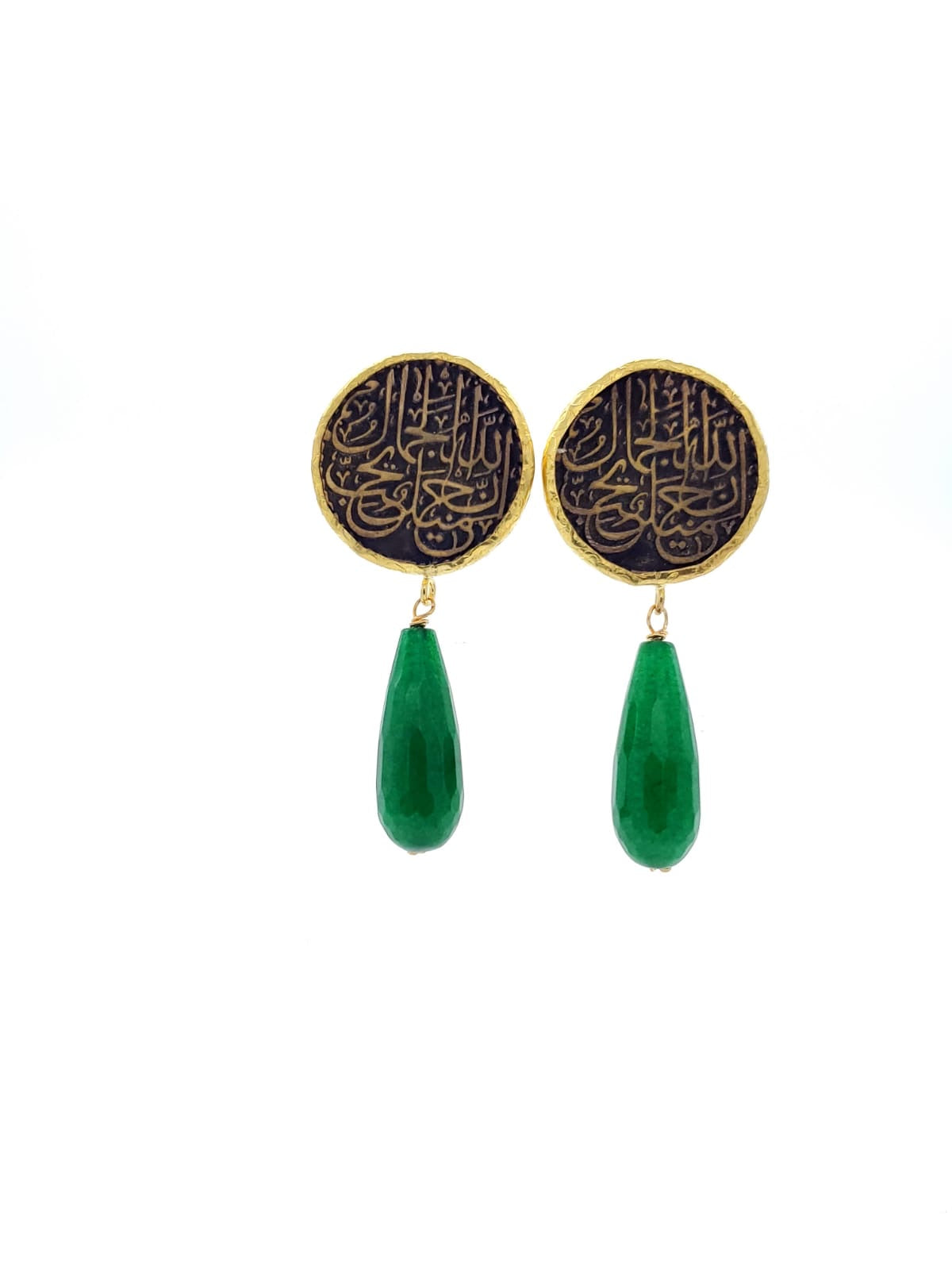This photograph features a pair of identical vintage-style earrings set against a pure white background. The central part of each earring is circular with a delicate gold outline, and an interior filled with intricate, squiggly designs in gold, set against a dark blue or bronze background. The designs, resembling Asian-inspired symbols, include a variety of shapes, many vertical and U-shaped, in differing sizes. Below each circular section, a gold latch and hook suspend a shiny, jade-colored teardrop, which exhibits a textured surface and darkens at the thicker base. These elegant earrings combine historical charm with intricate artistry, characterized by their dual-toned circular motifs and vibrant green dangles.